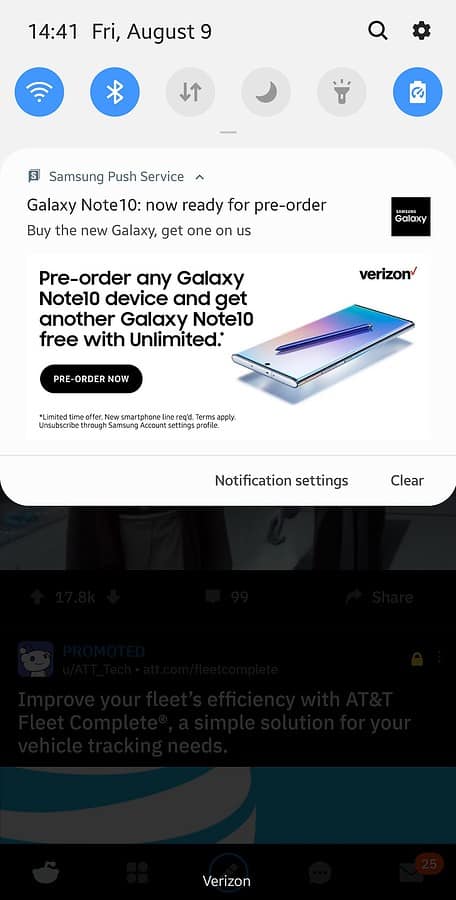This screenshot, taken at 14:41 on Friday, August 9th, on an Android phone, shows the top pull-down menu open on a Samsung device connected to Verizon. The notification center displays a message from the Samsung Push Service announcing that the Galaxy Note 10 is now available for pre-order with a special offer: buy one Galaxy Note 10 and get another one free with unlimited pre-order, exclusively through Verizon.

In the top menu, Wi-Fi and Bluetooth are enabled, while peer-to-peer sharing, night mode, and the flashlight are disabled. The battery saver is also visible but not activated.

Beneath the notification, the user is browsing the Reddit app. An advertisement for AT&T Fleet Complete, promoting a simple solution for vehicle tracking, is present. The footer of the phone screen confirms the Verizon carrier, and there is a Reddit post visible with 17,000 points, though its title is obscured.